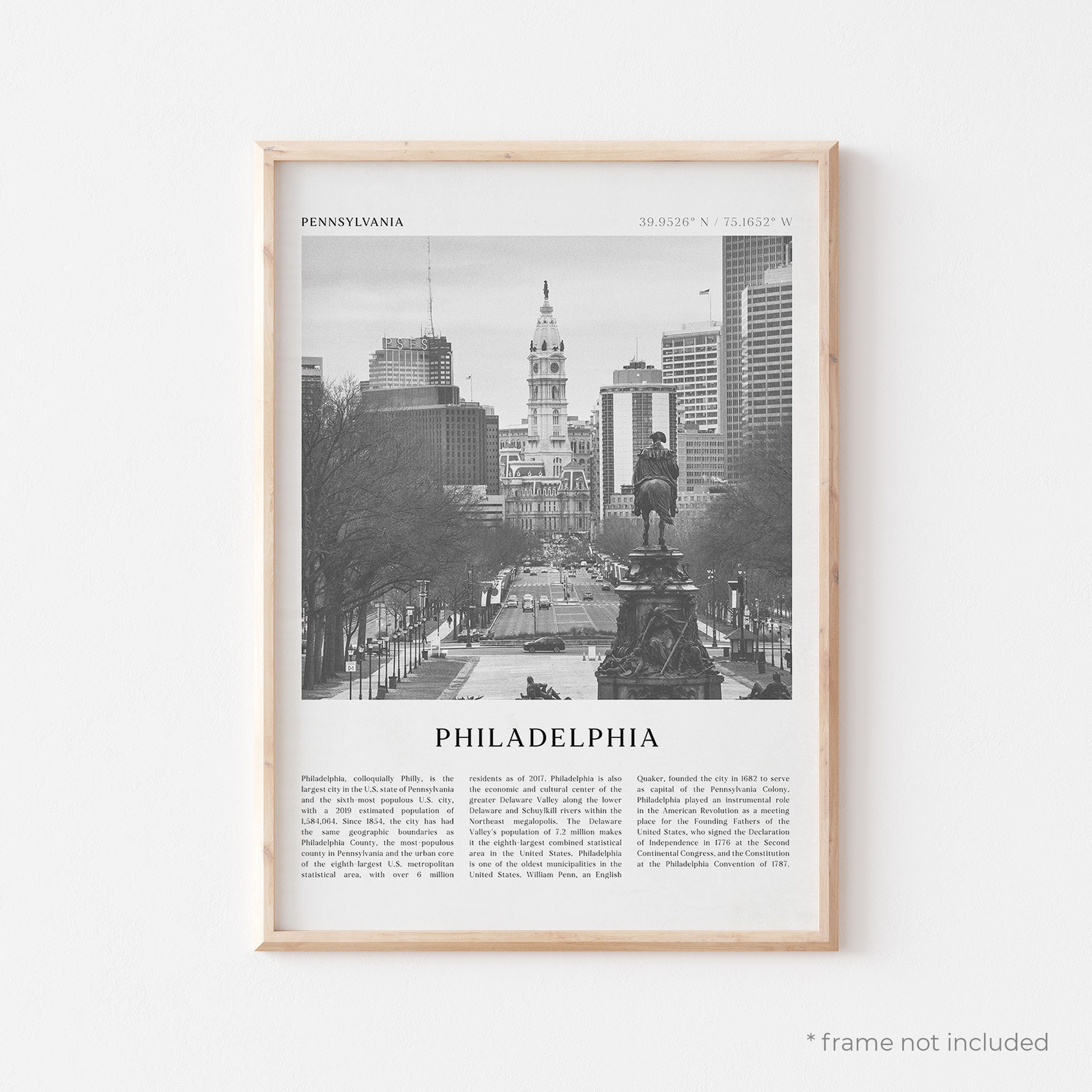The image is a framed black-and-white photograph from a news article or magazine, showcasing a historic scene of Philadelphia. The frame is made of very light-toned wood, enhancing the natural texture of the material. The article is titled "Pennsylvania" at the top left, with city coordinates on the top right. Dominating the center of the image is a well-known statue of a man on a horse, possibly Paul Revere, set amidst a bustling street lined with cars, trees, and pedestrians. Towering in the background is a prominent white building, likely Independence Hall, flanked by modern skyscrapers on either side. Sidewalks with lamps can be seen paralleling the street. At the bottom of the photograph is the city name "Philadelphia" in bold black letters, followed by a three-paragraph written passage detailing aspects of the city's profile, such as population and area. Notably, there's a message on the bottom right corner that reads "frame not included," in a subtle black-gray font.